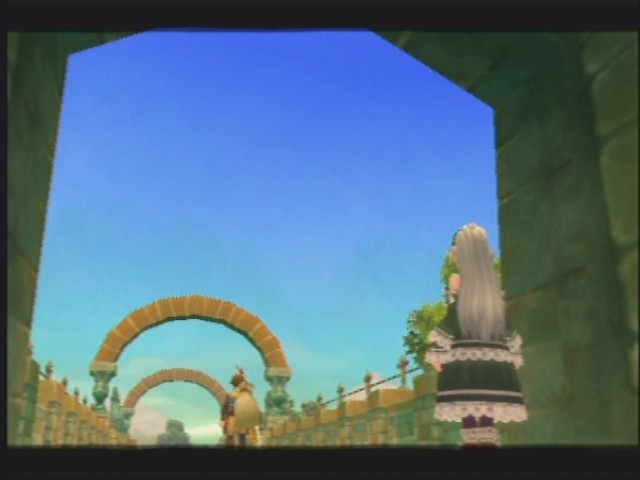The image appears to be a photograph of a TV screen displaying a screenshot from a video game. Captured with a camera, the photo showcases distinct television screen characteristics. The central focus of the scene is a female character with long, flowing grayish-silver hair and a gothic-style dress adorned with white frills and layers. She is dressed in purplish-red or possibly green leggings and appears to be looking away from the camera towards another individual whose gender and face are unclear, but is wearing yellow clothing. The setting features a brick bridge with multiple arches, and the characters are depicted standing under one of these arches with a clear blue sky visible through the arches in the background. The visual style of the game suggests simplicity, reminiscent of graphics from the early 2000s.